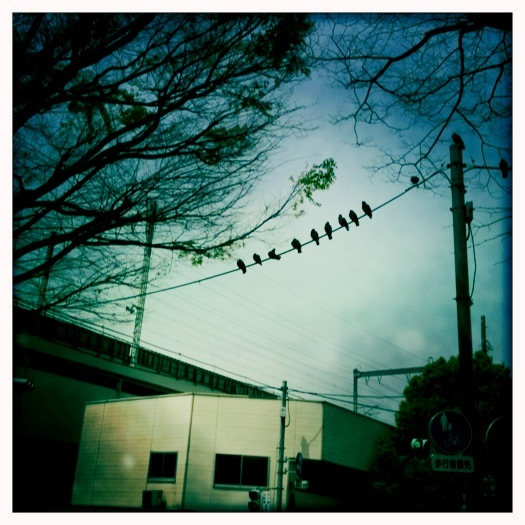This photograph, taken from a slight upward angle, captures a striking outdoor scene dominated by ten black birds perched in silhouette along a power line. The sky, a moody bluish-gray, suggests an overcast day, tinged with twilight. Below the wire lies an oddly-shaped white building, possibly a storage facility, nestled beneath an imposing bridge with additional cables arching across the sky. The landscape is framed by tree branches; to the left, greenery spills into the image, while the leafless branches to the right hint at fall or winter. In the bottom right corner, a shadowed and obscured pedestrian crossing sign adds a touch of urban life to the otherwise tranquil scene.